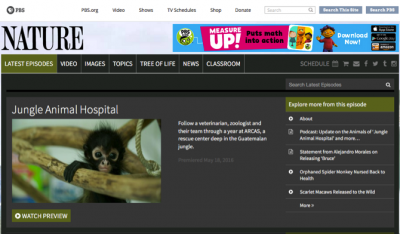The top section of the PBS Nature website is presented in a structured, user-friendly layout. At the top left corner, the PBS logo is prominently displayed, followed by six primary navigation buttons: PBS.org, Video, Shows, TV Schedules, Shop, and Donate. Adjacent to these buttons is a site search bar with the prompt "Search the site." This entire section features black text on a white background for clear visibility.

Beneath this navigation bar, the page features the title "NATURE" in bold, all-capital letters in black on a gray background. To the right of this title, a bright blue advertisement for a PBS game stands out, adding a splash of color to the otherwise muted tones.

Below this title section, a large, captivating image of a baby monkey immediately catches the eye. This adorable photograph is tagged with the text "Jungle Animal Hospital" just above it. Above this image, there is a secondary navigation bar comprising seven clickable options: "Latest Episodes" on a green background, and "Video," "Images," "Topics," "Tree of Life," "News," and "Classroom" on a black background with white text. 

To the right of these options, another button labeled "SCHEDULE" is accompanied by a series of clickable icons, enhancing the interactive nature of the site. 

Further down, users will find a dedicated search bar for browsing the latest episodes, followed by a green-highlighted call to action button labeled "EXPLORE MORE FROM THIS EPISODE." Below this button, additional clickable links are provided, guiding users to further content and information related to their current interests.